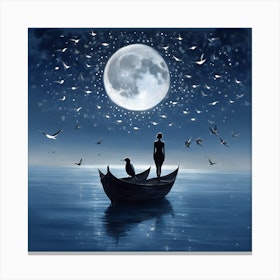The painting is a square-shaped, computer-generated image depicting a serene night scene. Dominated by shades of blue with touches of black and white, the bottom section of the painting features calm, dark blue water, faintly illuminated by a large, radiant moon overhead. A small rowboat, only large enough for a few people, floats on the water. Standing in the boat is a female figure, her back to the viewer, silhouetted against the moon's light. Beside her, on the edge of the boat, stands a sizeable bird with a long beak, also silhouetted. Additional birds, stylized and seemingly seagull-like, are seen flying around the moon, creating a sense of motion and life. The night sky, rich with stars, transitions from deep dark blue to slightly lighter hues towards the horizon. The entire scene exudes a tranquil yet captivating nocturnal atmosphere, with artistic highlights accentuating the details.